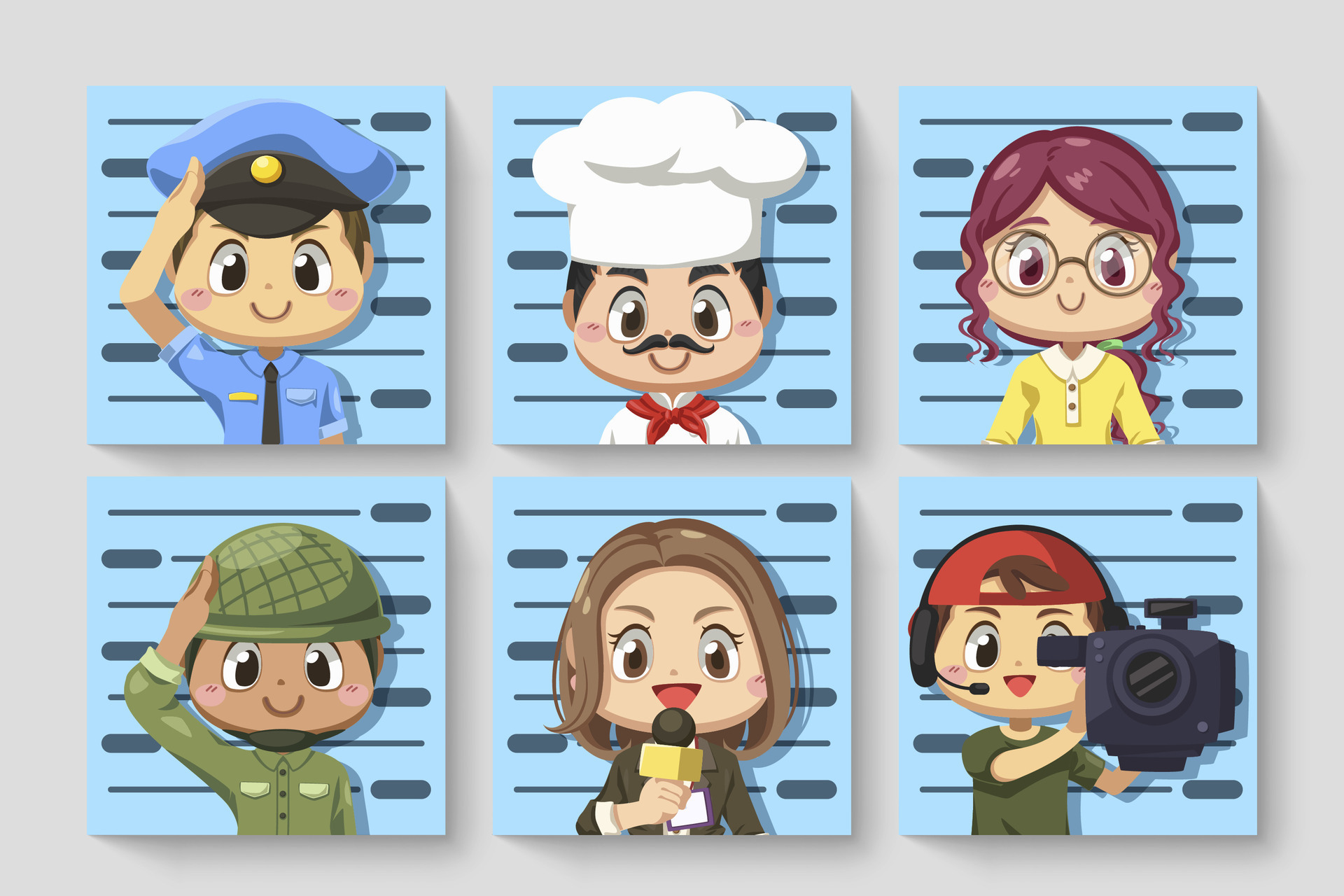This artistic image designed for a children's room features six square pictures, each depicting a different occupational character. Arranged in a neat grid of three on top and three on the bottom, these illustrations are presented within blue backgrounds and bordered by gray frames. The characters, each executed in a gouache style or CGI, boast distinct details that give them life.

Top left is a boy dressed as a policeman, saluting with a smile, donning a blue short-sleeved shirt, a blue hat with a black brim, and an insignia. Center top illustrates a male chef with black hair under a white chef's hat, a curled mustache, a red neckerchief, and a white chef's coat. The top right character appears to be a schoolteacher or librarian, portrayed as a woman with long brown curly hair tied back, wearing glasses and a yellow blouse with a white collar.

On the bottom left is a soldier, also saluting, dressed in olive green with a matching helmet. The middle bottom character is likely a news reporter, a woman with short brown bobbed hair holding a microphone, clad in a black suit with a press tag. Lastly, the bottom right image features a cameraman, a boy in a green shirt with a red cap worn backward, equipped with a camera and headphones with a microphone.

The overall image effectively conveys various career aspirations to inspire young minds. Each figure, characterized by their large oval eyes with expressive pupils and continuous smiles, contributes to an engaging and cheerful visual narrative.